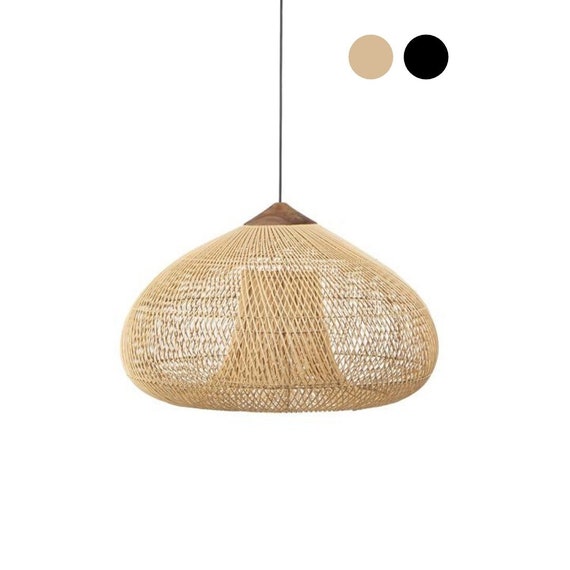The image features a hanging ceiling lamp with intricate detailing. The lamp's shade is crafted from straw-colored wicker woven into a pattern of small diamonds, creating a cross-woven texture that gives it a semi-transparent, net-like appearance. The weaving folds upward towards the center, forming a flat-topped cylindrical structure beneath the fixture. The top of the lamp features a dark brown, pyramid-shaped wooden piece that connects to a slender, dark brown cord or wire, from which the lamp is suspended against a plain white background. On the upper right side of the image, two circular color options are displayed: a smaller circle on the left showing the current straw color of the lampshade, and a larger circle on the right indicating a black color option. The overall structure of the lampshade resembles a teardrop or Hershey's Kiss shape, highlighting the elegance and versatility of the rattan material used in its design.